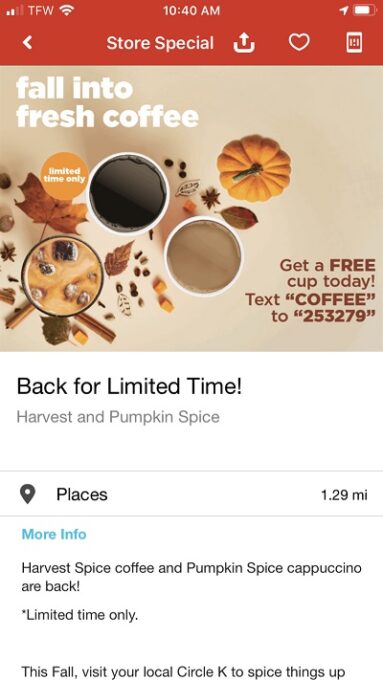The image features a smartphone screen with the following elements detailed in order:

- **Top Section**: The screen is bordered in red and displays a signal strength of 2 out of 4 bars with the "TFW" carrier label on the top left. The time reads 10:40 AM and the battery shows approximately 80% charged. Below the status bar is an icon indicating a less-than symbol alongside text that reads "Store Special."

- **Action Icons**: Following this, there are several action icons: a forward arrow, a heart, and an unspecified icon.

- **Middle Section**: The advertisement prominently features two paper cups – one filled with black coffee and the other containing coffee with some added creamer. Positioned next to these cups is a glass of iced coffee decorated with ice cubes. The scene is further accentuated with a piece of cinnamon, fall leaves, and a miniature pumpkin.

- **Promotional Text**: The message "Get a free cup today" is shown, prompting users to text "COFFEE" to the number 253279. Beneath this, additional promotional text reads: "Back for a limited time, Harvest and Pumpkin Spice. Distance: 1.29 miles. More info: Harvest Spice Coffee and Pumpkin Spice Cappuccino are back, limited time only."

- **Footer**: The concluding call to action encourages readers with, "This fall, visit your local Circle K to spice things up."

This comprehensive caption vividly captures the promotional content and festive imagery of a limited-time coffee offer at Circle K.